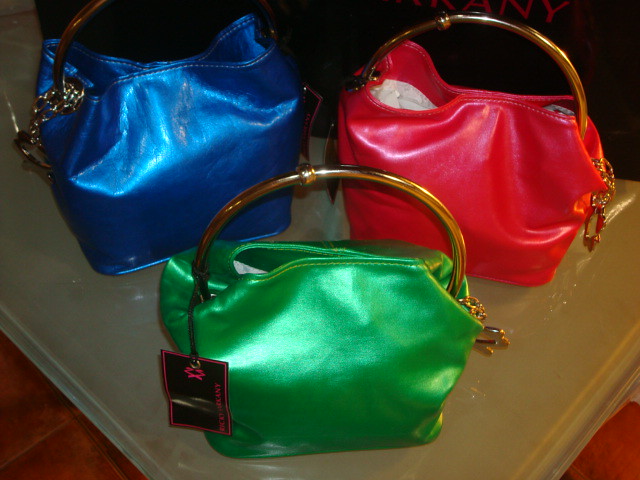The image depicts a display of three vibrant ladies' handbags positioned on a shiny white table, which rests upon a reddish-brown wood floor. Each handbag is crafted from a highly reflective material, possibly suede, leather, or a metallic fabric that gives off a high sheen, enhancing their eye-catching appearance.

To the upper left of the table is a blue handbag featuring a curved gold handle and a matching gold chain. Adjacent to it on the upper right is a pinkish-red handbag, also equipped with a curved gold handle and a gold chain on its side. The handbag at the bottom is lime green, showcasing the same gold handle, gold chain, and an additional gold zipper with a small keychain attached to the side. This green bag also has a noticeable black tag with pink lettering, which is also seen on the red handbag, though the specifics of the lettering are unclear.

The red handbag appears to be stuffed with packing material to maintain its shape for display purposes. Despite the flash being used, the overall lighting conditions make it difficult to capture finer details, suggesting the photo was taken in less-than-ideal lighting.